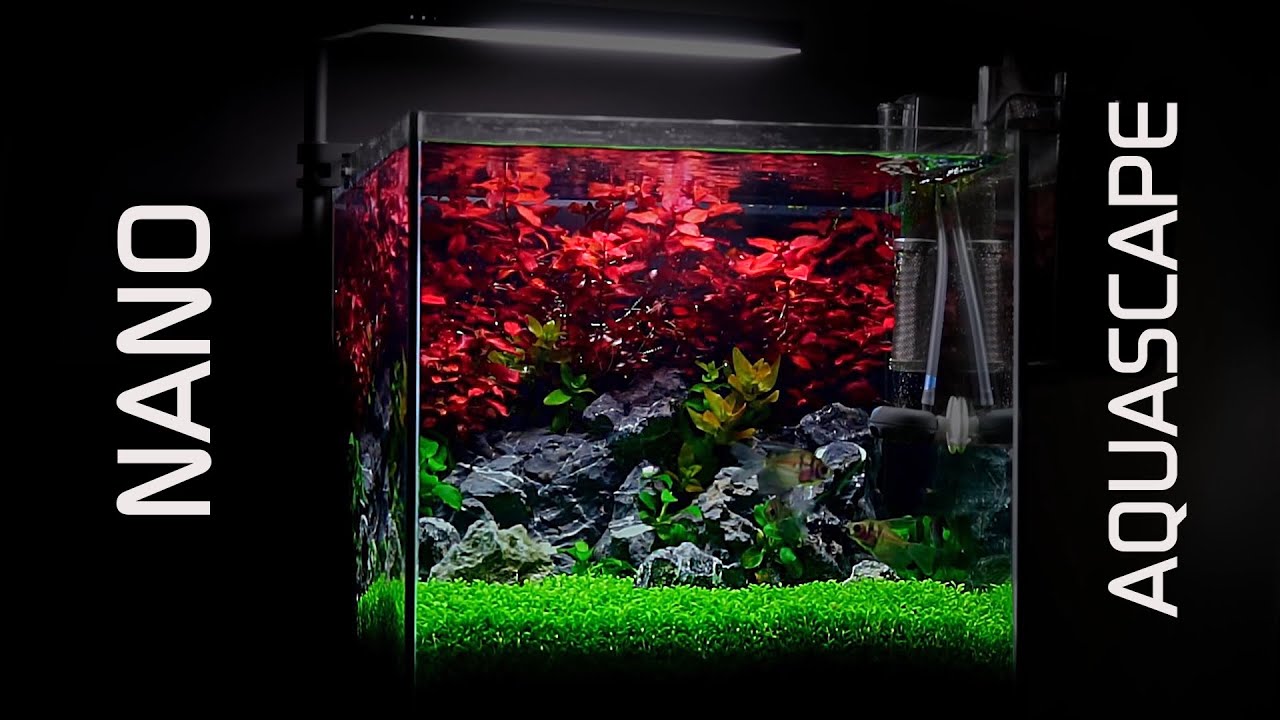The image features a fish tank showcased against a black background. The words "NANO" and "AQUASCAPE" are written vertically in white capital letters on the left and right sides of the image respectively, both from bottom to top. Positioned centrally, the glass tank is illuminated by a long light fixture seemingly attached to its left side. Inside, the tank is filled with water, and the bottom is covered in a green substrate. The aquascape includes gray rocks and plant life, with red flowers adding a pop of color. Additionally, tubes are visible on the right-hand side of the tank, enhancing the intricate aquatic setup. There are no fish in the tank.